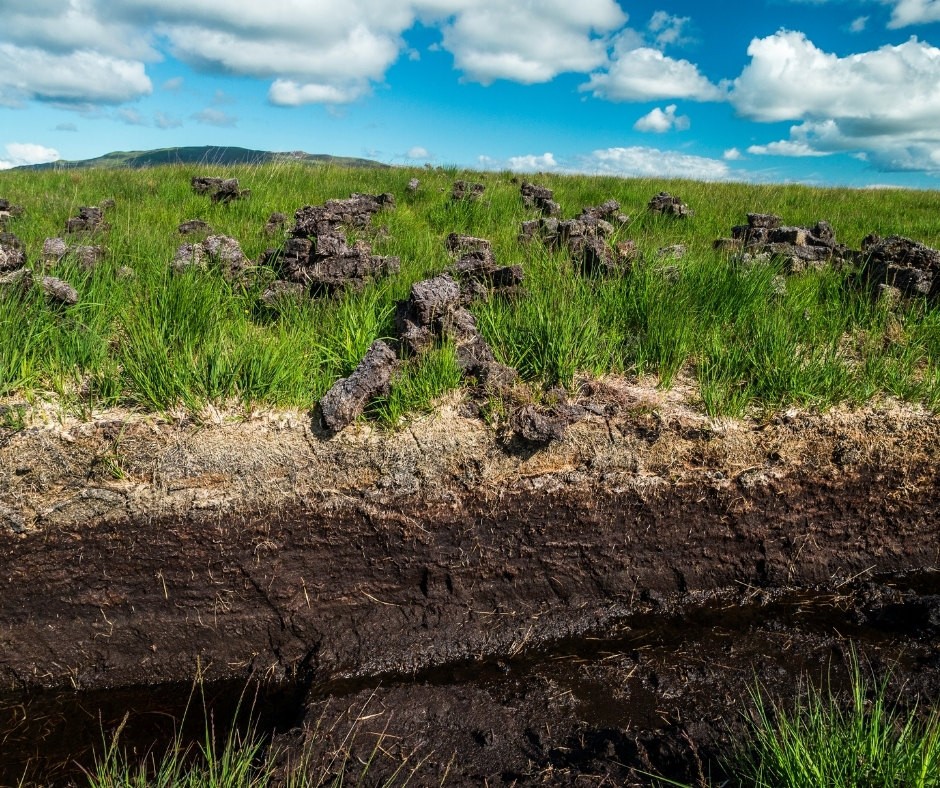The image captures a detailed landscape featuring a rock and mud outcropping with a recent wet surface that is drying out. At the forefront, the earth forms a steep edge where green grass transitions sharply before continuing on top. Scattered across the grass are multiple mounds of dark brown and black rocks that appear almost geometric, giving the impression of ancient ruins. The sky is a vivid blue, dotted with large, fluffy white clouds, providing a well-lit backdrop. In the distance, there is a small mountain range visible in the top left corner. The overall scene conveys a lush and vibrant environment, with professionally taken quality and no text overlay.